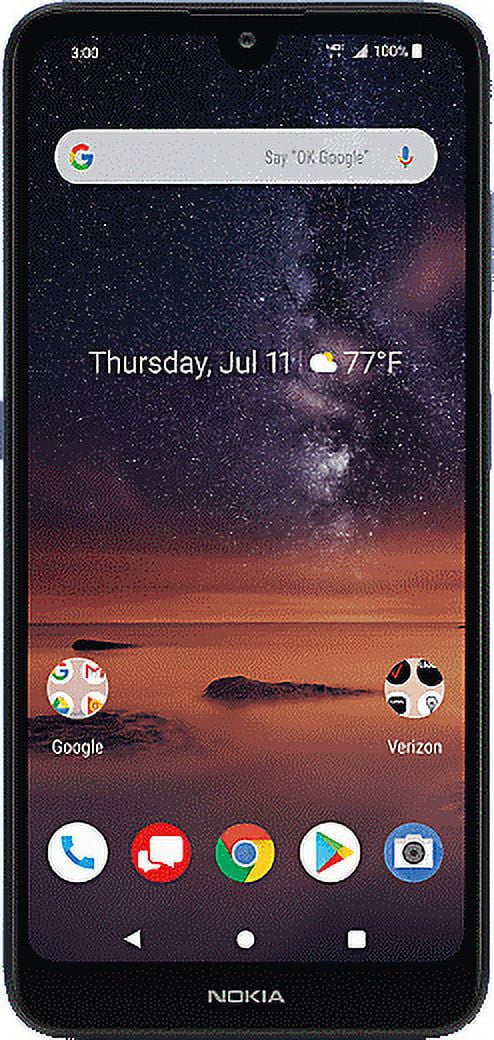This image captures a Nokia smartphone displaying a user’s home screen. Prominently, the screen is adorned with a starry night backdrop set in a desert landscape. At the bottom, the brand "Nokia" is clearly visible. The home screen showcases a neat arrangement of app icons and widgets. From right to left, the primary row of icons includes the Phone, Messaging, Chrome, Google Play, and Camera apps. Additionally, there are two folder icons holding multiple apps; the one on the right labeled "Google" contains a variety of Google services, and the one on the left labeled "Verizon," possibly housing essential service apps.

Above these icons, on the right-hand side, a weather widget indicates it is Thursday, July 11th, with a temperature of 70 degrees Fahrenheit. The weather is slightly cloudy, as depicted by a sun peeking out from behind a cloud. Centered above this widget is the Google Search bar, making search functionality easily accessible. At the top of the screen, the status bar displays the time as 3:00 PM, a full 4G signal, and a fully charged battery at 100%.